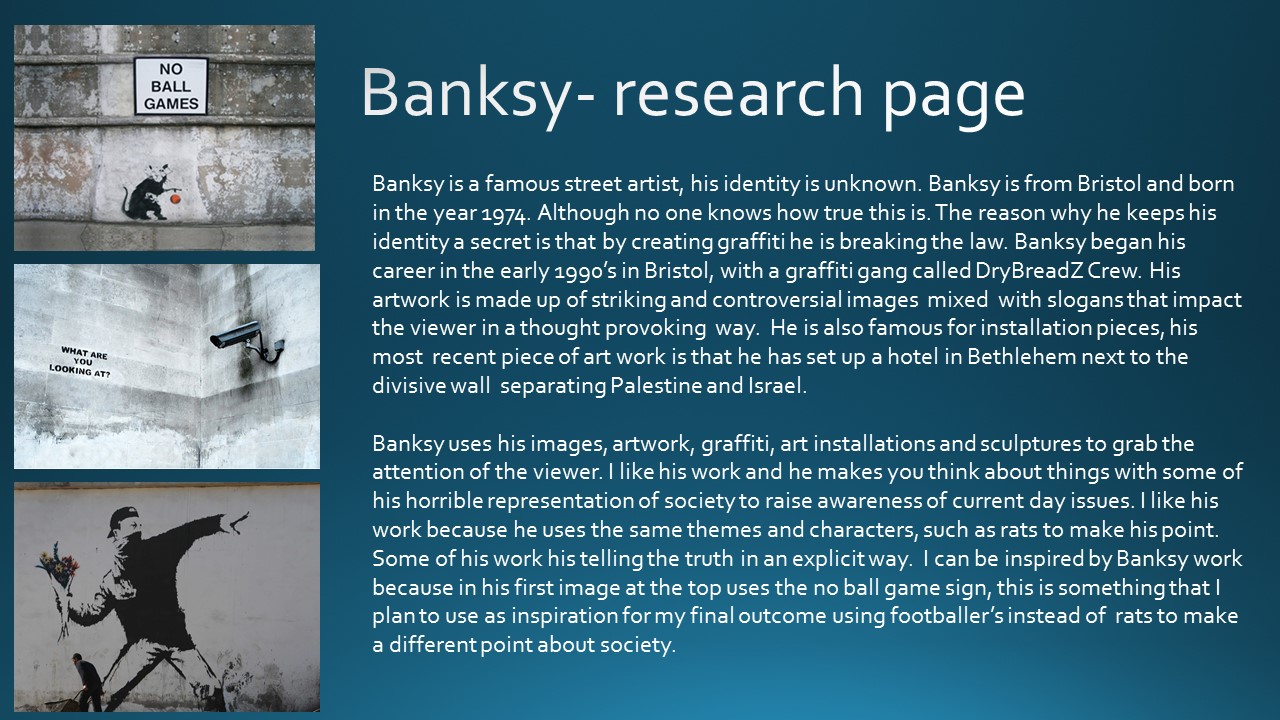This image features a blue background with the title "Banksy Research Page" written in white at the top. On the left side of the image are three black and white illustrations. The top illustration depicts a rat dribbling a basketball alongside text that reads "No ball games." The middle illustration shows a surveillance camera mounted on a wall, pointing toward the phrase "What are you looking at?" The bottom illustration portrays a baseball player, about to pitch, but instead of a ball, he holds a bouquet of flowers. A figure is cleaning behind him, adding an element of mystery to the scene.

On the right side of the image, extensive text provides information about Banksy, noting that he is a famous street artist from Bristol, born in 1974, though his identity remains unknown. The text explains that Banksy's anonymity is crucial as his graffiti work is illegal. Originating in the early 1990s with the graffiti gang Dry Bread Z Crew, Banksy's art combines striking, controversial images with impactful slogans. His works often aim to provoke thought and raise societal awareness, using recurring themes and characters such as rats. Additionally, Banksy is known for his installation pieces, including a notable recent project set up in a hotel in Bethlehem next to a wall separating Palestine and Israel.